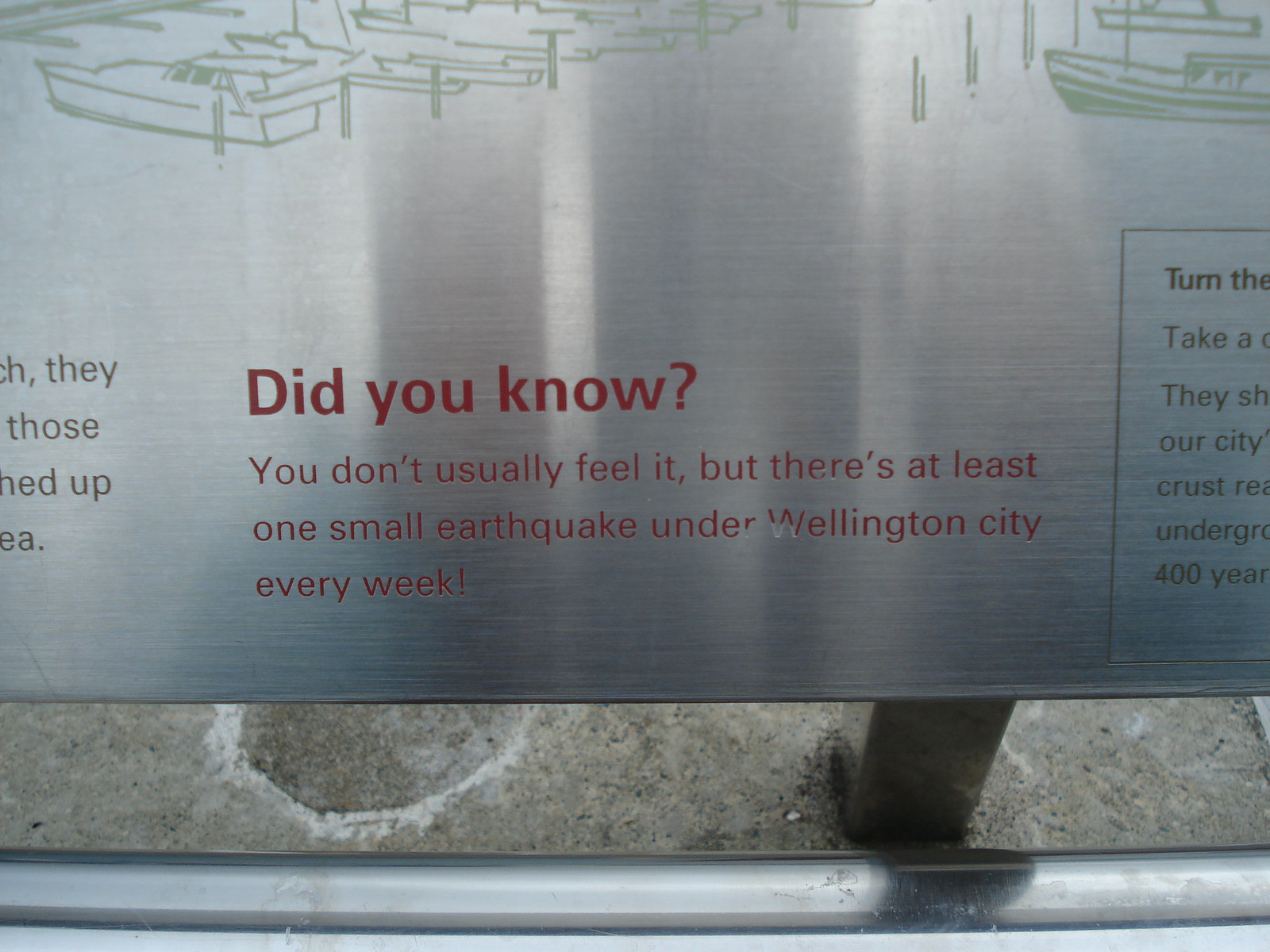This image captures the lower portion of a shiny, silver metal information sign, installed in a concrete sidewalk post. The sign's upper part is adorned with green line drawings of various boats docked, although this section is partly cut off by the camera. Prominently displayed in the middle of the sign, in bold red text, is the heading "Did You Know?" followed by the message, "You don't usually feel it, but there's at least one small earthquake under Wellington City every week." To the left and right of this red text, additional black lettering is visible but partially obscured, with discernible fragments such as "they", "our city", and "400 year." The brushed metal surface of the sign has subtle white streaks, adding to its reflective appearance. At the base of the sign, a steel pole is also visible.